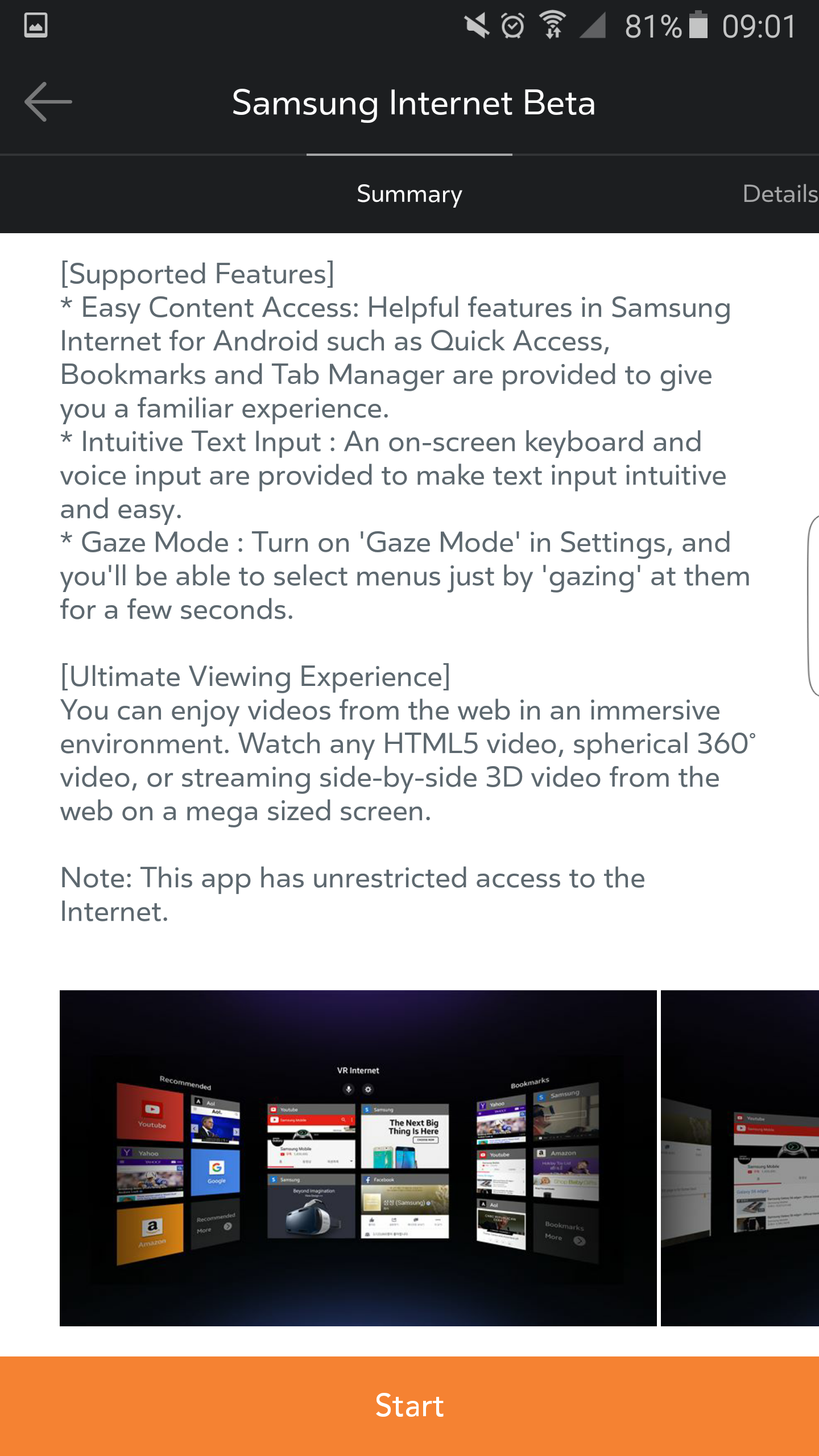This image is a screenshot showcasing an informative page about the Samsung Internet Beta browser. In the upper right corner, it displays the time as 9:01, the battery level at 81%, active Wi-Fi connection, and an alarm clock icon, all set against a black background. The main content is divided into two sections: 

1. On a white background, there's a heading labeled "Supported Features," followed by a series of detailed descriptions:
   - **Easy Content Access:** Highlights the helpful features available in Samsung Internet for Android, including quick access, bookmarks, and a tab manager, designed to offer a familiar browsing experience.
   - **Intuitive Text Input:** Explains that the browser provides an on-screen keyboard and voice input to ensure text entry is straightforward and user-friendly.
   - **Gaze Mode:** Describes a feature where users can enable "Gaze Mode" in settings, allowing them to select menu items by gazing at them for a few seconds.
   - **Immersive Video Watching:** Describes the immersive environment offered when watching videos from the web, including support for HTML5 video, spherical 360-degree video, or side-by-side 3D video on a large screen.

2. Against the black background, there's a header for "Samsung Internet Beta" with a summary arrow pointing left located in the lower right corner.

The visual layout emphasizes accessibility and ease of use, detailing innovative features designed to enhance the browsing experience on Samsung devices.